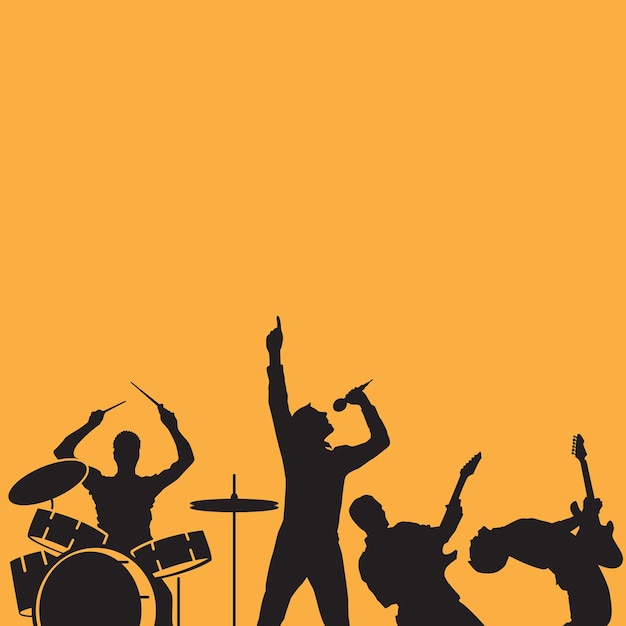This illustration, set against a warm peachy-orange background, vividly depicts a musical band in silhouetted form. Featuring four band members, their dynamic poses convey the energy and passion of their performance. On the left, the drummer stands poised with both hands raised, drumsticks aimed at a full drum set with visible cymbals. Next to him, the singer grips a microphone in his right hand, his left index finger pointed skyward as he prepares to belt out a note. To the singer's left, one guitarist stands firm, guitar neck extended outward as he rocks out. Further to the left, another guitarist is captured in mid-action, dramatically bending backward, his guitar positioned vertically as he jams. The black silhouettes against the striking background emphasize the theme of music and movement in this two-color illustration.